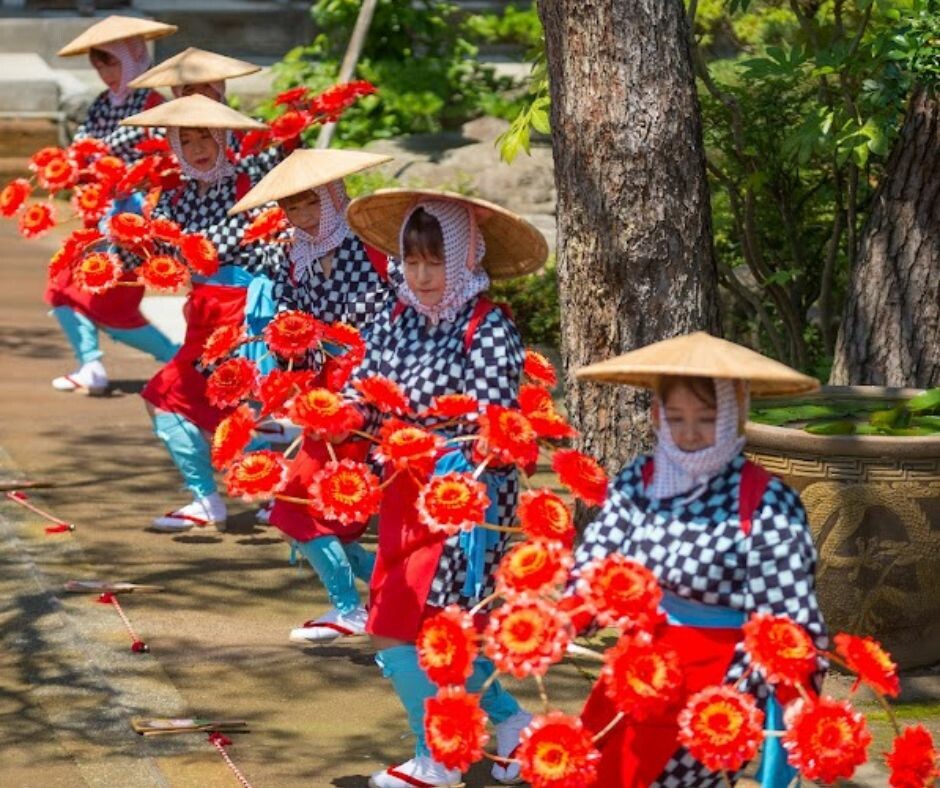The vibrant color photograph, taken in landscape orientation, showcases a group of six Asian women standing in a diagonal line from the top left to the bottom right of the image. Each woman is adorned in a pointed, light brown or beige straw hat, complemented by white headscarves with stripes tied under their necks. Their outfits consist of black and white checkered tops with a touch of red scarf draped over their shoulders, neatly fastened with an aqua blue sash. They wear aqua or turquoise colored pants, white socks, and red flip-flops. Each woman holds a cluster of red flowers, arranged on sticks that together resemble a small parasol, adding an elaborate touch to their appearance. In addition to the detailed attire, the background features lush green foliage and tall tree trunks with brown bark, all set upon a gray cement floor. The women appear engaged, looking around and at each other, contributing to the image's realistic and representational style.